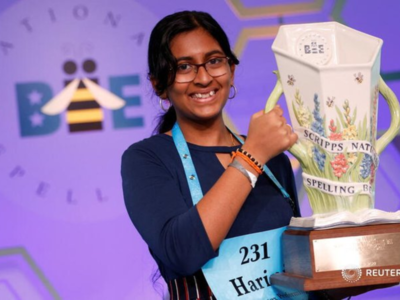The photograph captures a woman with black hair and glasses, smiling broadly. She is adorned with silver hoop earrings and various bracelets, including gray and white, orange, and black and yellow striped ones. The woman is wearing a dark blue dress and a sky blue name tag around her neck, which reads "231 Harry." She holds a distinct trophy featuring a white cup at the top and a brown wooden base, decorated with green vegetation, flowers, and bees. The trophy bears the inscription "Scripps National Spelling Bee." Behind her, the background is predominantly purple, with a board displaying the text "Bee," where the middle "E" is creatively styled using the shape of a bee. Honeycomb patterns and additional bee motifs enhance the thematic speller's victory scene.